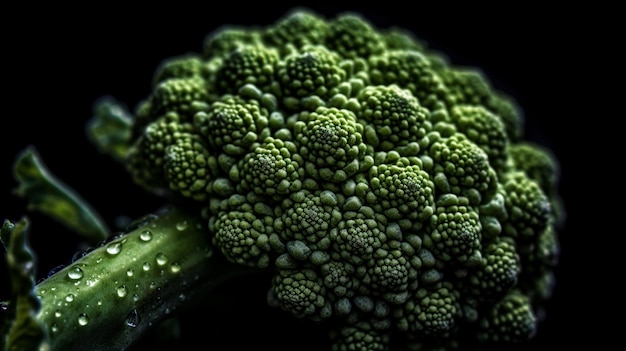This close-up photograph captures the intricate details of a broccoli head against a pitch-black background. The central focus is on the densely packed, bead-like clusters of the broccoli florets, which exhibit a bumpy texture and vary in size. The dark green florets, coupled with the dark green leaves, create a rich, verdant scene, highlighted by glistening water droplets that resemble pearls. These droplets add a sense of freshness and realism to the image, shimmering under the light. The angular, green stem and surrounding leaves appear in the lower left and background, slightly blurred to emphasize the central florets. Despite its realistic appearance, the photograph's sharp detail and texture give it an almost surreal, computer-generated quality, making the broccoli seem like an alien landscape or a meticulously crafted graphic.